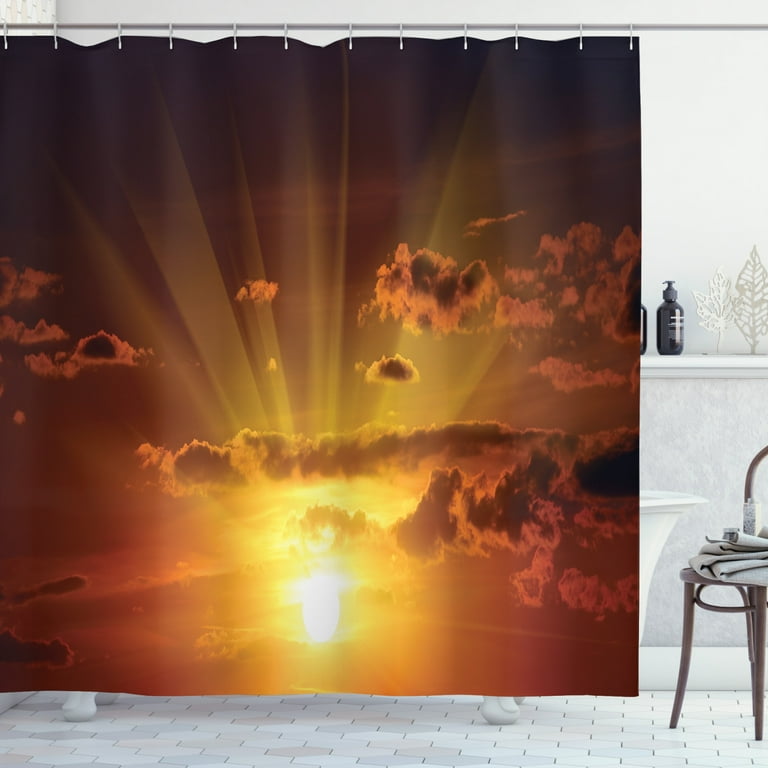This image captures a serene bathroom setting, dominated by a striking shower curtain depicting a vibrant sky transitioning from sunset to night. The curtain is adorned with hues of brown and yellow, showcasing a bright sun with its rays illuminating the clouds in shades of brown and orange, giving the appearance of a glowing sky. The white clawfoot bathtub, partially visible at the bottom and right side, is accompanied by a metallic chair with gray legs and a white seat, holding neatly folded towels. To the right of the tub, a shelf displays gray shampoo bottles, while decorative white tree statuettes add a touch of elegance to the ledge above. The bathroom is characterized by its pristine white tiles and painted walls, creating a calm and clean atmosphere.